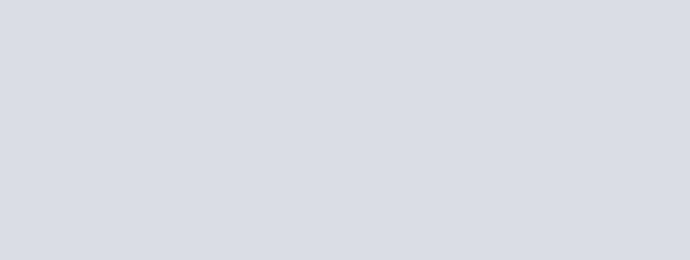The image depicts a screenshot featuring a blank page with a subtle gray gradient background. The gradient progresses diagonally from the bottom left to the top right, blending from a light gray at the bottom to a medium gray at the top right. The bottom of the page appears to have a length approximately between 8 to 15 inches, while the width is estimated to be around 4 inches. This creates a smooth, minimalist appearance with a diagonal gradient transitioning from lighter to darker tones.